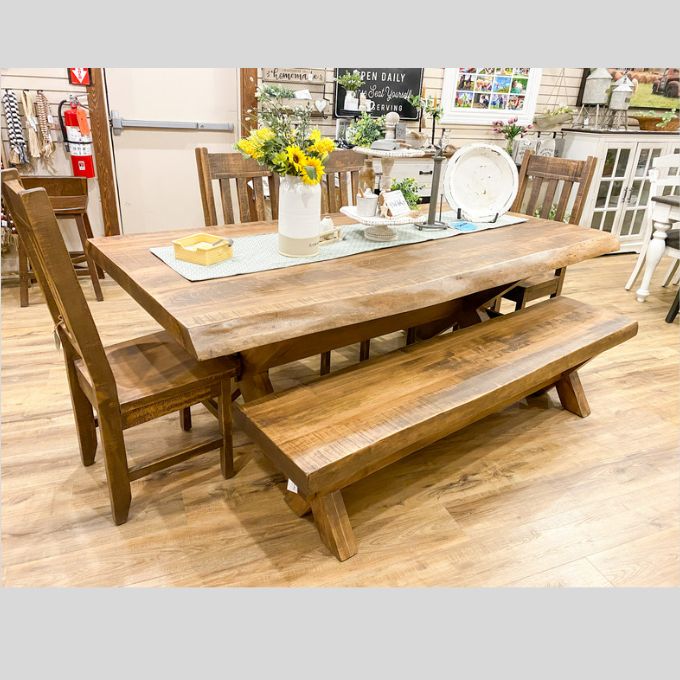This is a color photograph taken inside what appears to be a public restaurant or store specializing in household goods, as suggested by the sign indicating "open daily" and various public features like a push-handle door and a fire extinguisher. The focal point is a large dining room table, striking because of its notably thick, unfinished wood, measuring approximately four to five inches in thickness. The table is surrounded by four wooden chairs of the same material and a long wooden bench on one side. The table is set on a wooden floor, topped with a white runner that hosts several objects: a plate on a stand, a paper towel holder, and a white jug filled with yellow daisies and baby breaths. There’s also a suggestion box, a greeting card, and a star on a pedestal adding to the display. In the background, a white cabinet holds a model of water tanks, contributing to the overall ambiance. Although other objects are visible in the background, they are too far away to be distinctly identified, hinting at a spacious, open setting, possibly extending into a kitchen area.